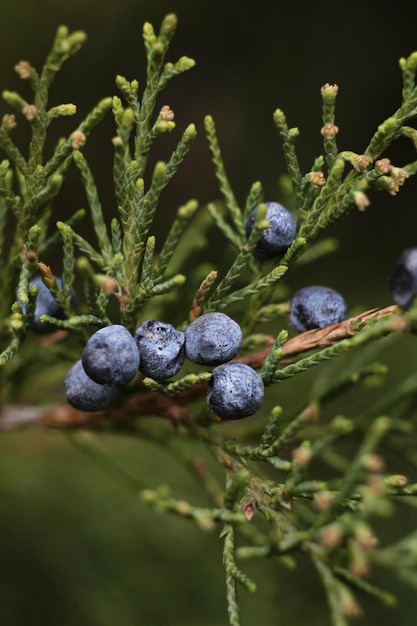Close-up portrait photograph capturing the intricate details of juniper berries. The image is sharply focused, highlighting both the texture and vibrant color of the juniper leaves and berries. The juniper leaves, resembling reptilian scales, are green with a hint of dryness, and the tiny needles are meticulously detailed. Dominating the center-left of the image are five prominently displayed berries, resembling shriveled purple wine grapes, with a rich purple hue indicating their ripeness. A brown stem stretches horizontally across the frame, adding an organic element to the composition. Additional berries can be seen in the background on the left and the top right, slightly out of focus but still contributing to the overall natural ambience. The photograph captures the beauty in the small-scale details of nature.